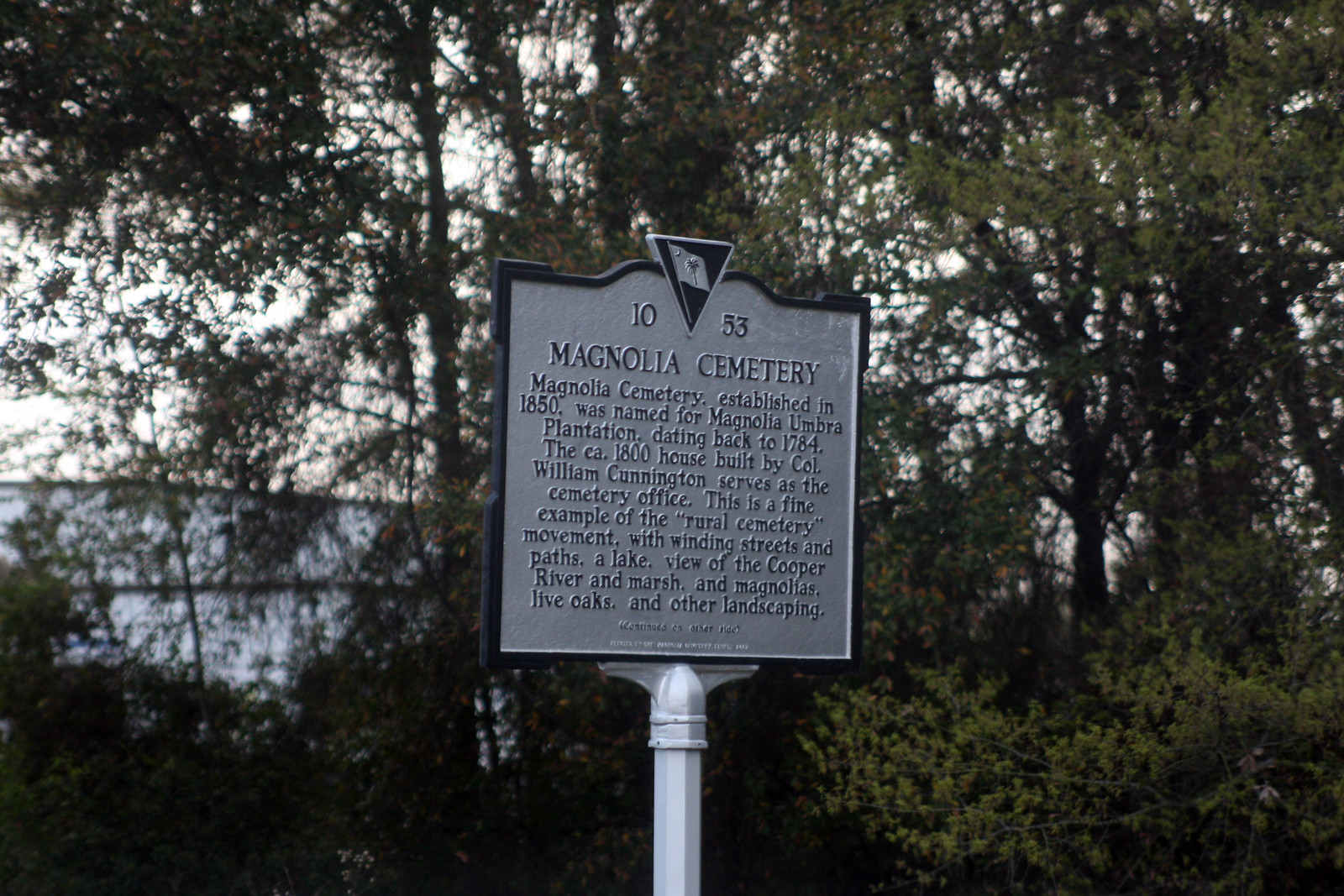An iron sign with a black border and white background stands on a white metal post in front of Magnolia Cemetery. The top of the sign features an upside-down triangle with a black background and a white inset flag, likely the flag of South Carolina. To the left of the triangle is the number "10," and to the right, "53". The sign prominently displays the name "Magnolia Cemetery." Below, the text reads: “Magnolia Cemetery, established in 1850, was named for Magnolia Umbra Plantation, dating back to 1784. The CA 1800 home, built by Colonel William Cunnington, serves as the cemetery office. This is a fine example of the rural cemetery movement, featuring winding streets and paths, a view of the Cooper River and marsh, and landscaping with magnolias, live oaks, and other flora." In the background, tall trees, short shrubs, and a building can be seen.